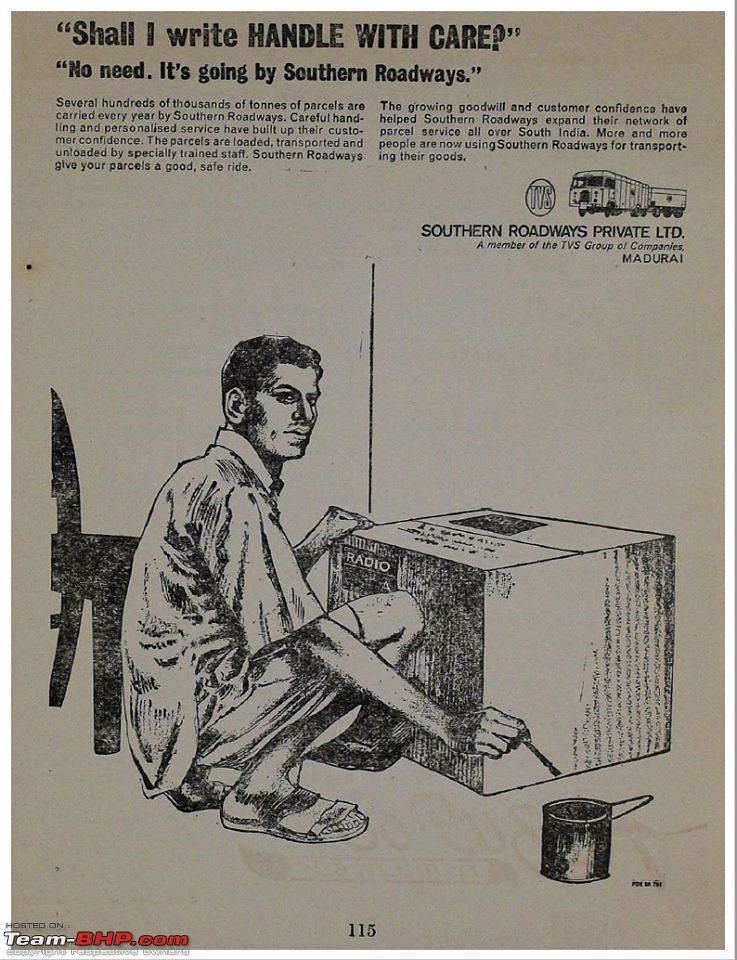This image is an advertisement for Southern Roadways, depicting a pencil drawing of a man preparing a package. The man, dressed in a short-sleeved shirt, shorts, and flip flops, is seen kneeling beside a box, applying a label with a small paintbrush and a can of paint beside him. A chair is visible nearby. At the top of the image, the text reads, "Shall I write 'Handle with care'?" followed by, "No need, it's going by Southern Roadways." The advertisement emphasizes the company's meticulous handling and personalized service, stating that several hundreds of thousands of tons of parcels are carried annually. Southern Roadways' specially trained staff load, transport, and unload parcels, which ensures a safe ride and has built strong customer confidence. Additionally, the growing goodwill has allowed Southern Roadways to expand their parcel service network across South India. The company's name, Southern Roadways Private LTD, is noted at the bottom of the image, alongside a small depiction of a Southern Roadways truck. The image also includes a reference to "page 115," suggesting it may be part of a magazine or similar publication.